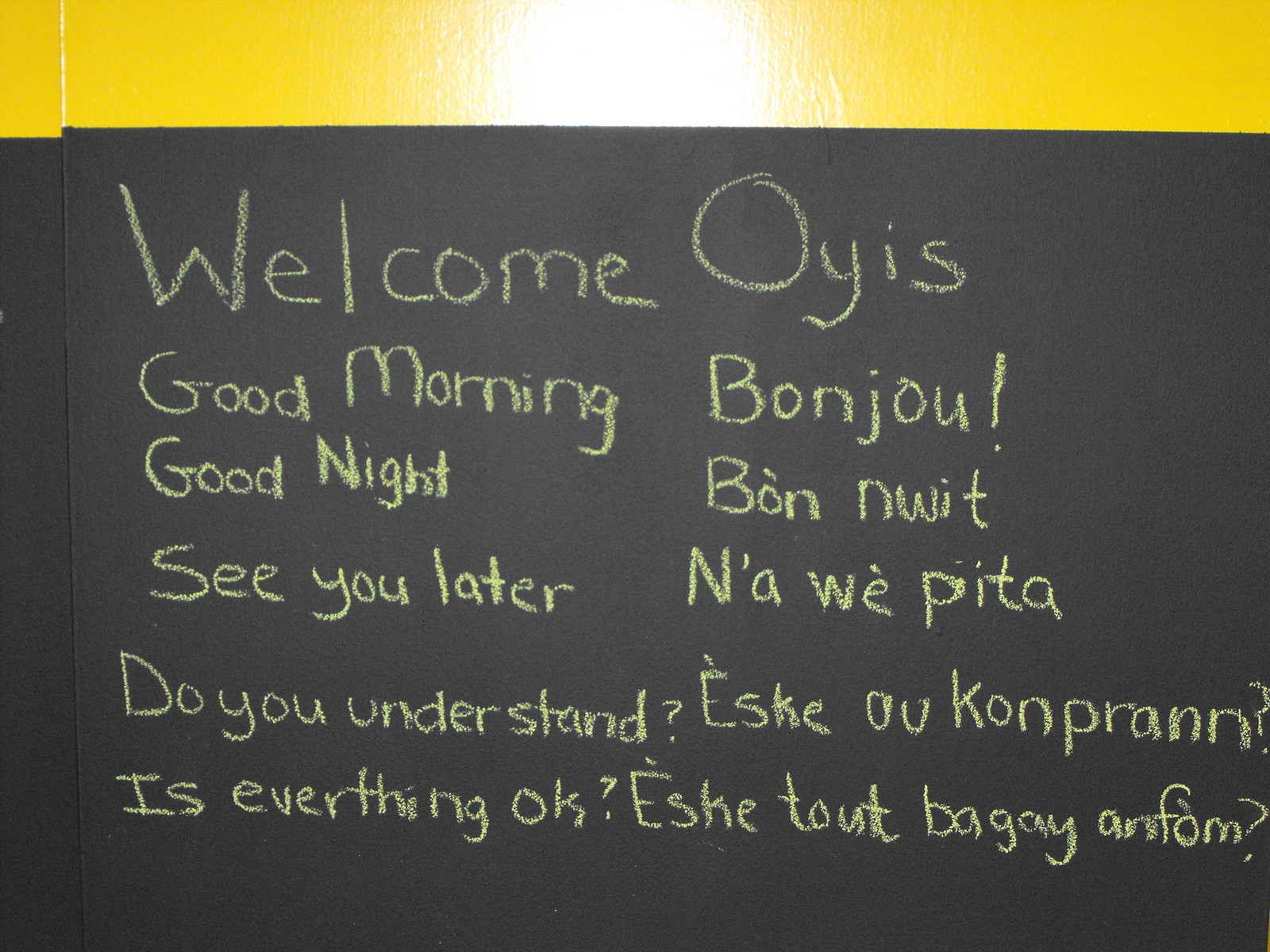The image is a color photograph in landscape orientation, depicting a blackboard with handwritten text in yellow chalk. At the top of the blackboard, there is a shiny yellow strip that has a white circular glow. The majority of the blackboard is filled with phrases written in yellow chalk, horizontally across the black surface. The left side of the board features text in English: "Welcome," "Good Morning," "Good Night," "See You Later," "Do You Understand," and "Is Everything Okay?" Each phrase is mirrored in a foreign language on the right side of the board, with translations such as "OYAS," "Bonjour," "Bon Nuit," "nawipita," "Es que o comprend," and "Es que tu page inform." The text appears to be set in a realistic, handwritten chalk typography style. The photograph captures the subject in a representational manner, making the handwritten chalk text on the blackboard the focal point of the image.